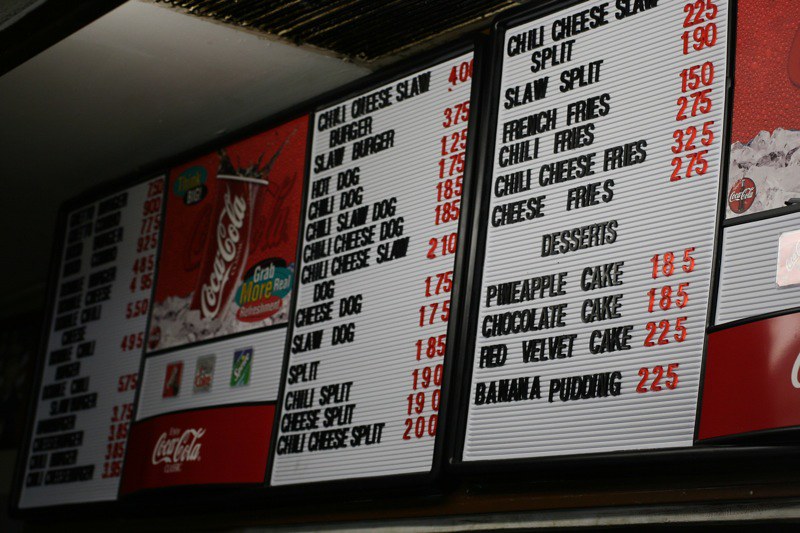The menu prominently displays a Coca-Cola advertisement in the center, indicating the sponsorship with additional Coca-Cola branding elements. The background of the menu is white, with prices marked in distinct red numerals and descriptions of items in black lettering. This menu, designed to be mounted on a wall, primarily features a variety of hot dogs and related items. Central to the offering are items such as a chili cheese slaw burger, slaw burger, hot dog, chili dog, chili slaw dog, chili cheese dog, chili cheese slaw dog, cheese dog, slaw dog, and a variety of “split” items including chili split, cheese split, and chili cheese split. They also offer a range of fries – plain, chili fries, chili cheese fries, and cheese fries. Sweets round off the menu with a selection of desserts including pineapple cake, chocolate cake, red velvet cake, and banana pudding. A Coca-Cola paper cup filled with ice cubes is also showcased on the menu, emphasizing the beverage choice.